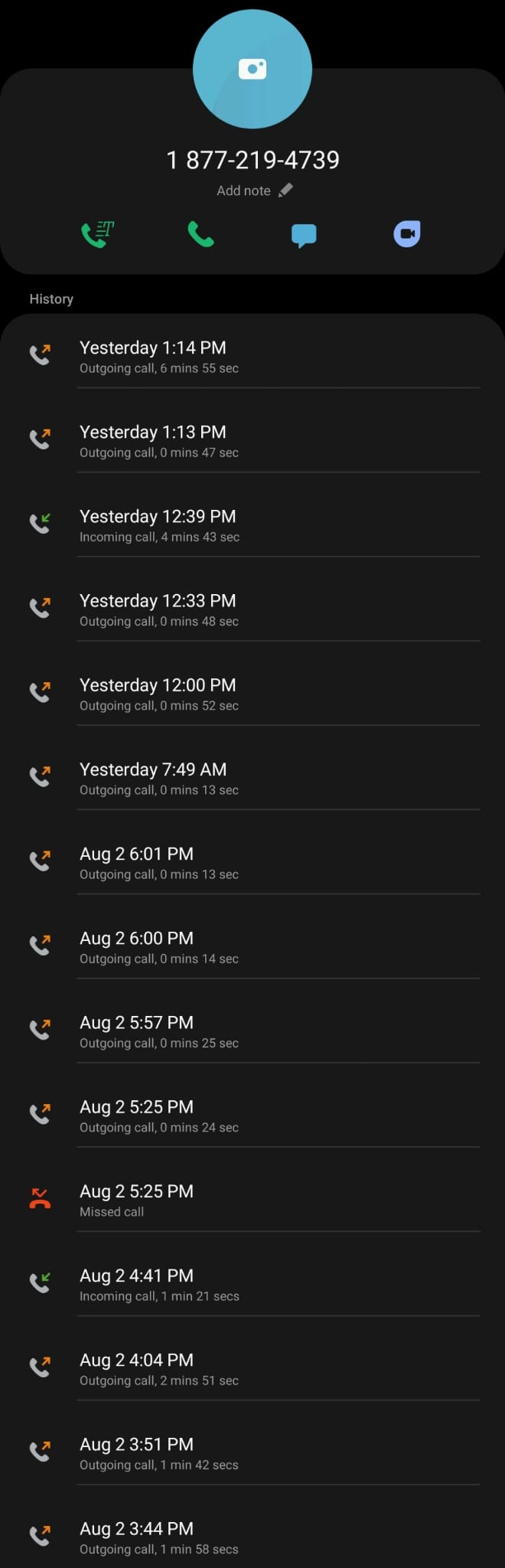The image is a screenshot of a cell phone's call log with a black background. At the top, there is a blue circle featuring a white camera icon in its center. Below this icon, the phone number "1-877-219-4739" is displayed, alongside an "add note" option. The phone interface includes a green telephone handset icon with a 'T' above it, a separate green handset icon, a blue text message bubble icon, and a blue teardrop-shaped icon with a black video camera symbol inside.

The call history is detailed chronologically as follows:

- **Yesterday**
  - **1:14 p.m.:** Outgoing call lasting 6 minutes and 55 seconds.
  - **1:13 p.m.:** Outgoing call lasting 47 seconds.
  - **12:39 p.m.:** Incoming call lasting 4 minutes and 43 seconds.
  - **12:33 p.m.:** Outgoing call lasting 48 seconds.
  - **12:00 p.m.:** Outgoing call lasting 52 seconds.
  - **7:49 a.m.:** Outgoing call lasting 13 seconds.

- **August 2nd**
  - **6:01 p.m.:** Outgoing call lasting 13 seconds.
  - **6:00 p.m.:** Outgoing call lasting 14 seconds.
  - **5:57 p.m.:** Outgoing call lasting 25 seconds.
  - **5:25 p.m.:** Outgoing call lasting 24 seconds.
  - **5:25 p.m.:** Missed call.
  - **4:41 p.m.:** Incoming call lasting 1 minute and 21 seconds.
  - **4:04 p.m.:** Outgoing call lasting 2 minutes and 51 seconds.
  - **3:51 p.m.:** Outgoing call lasting 1 minute and 42 seconds.
  - **3:44 p.m.:** Outgoing call lasting 1 minute and 58 seconds.